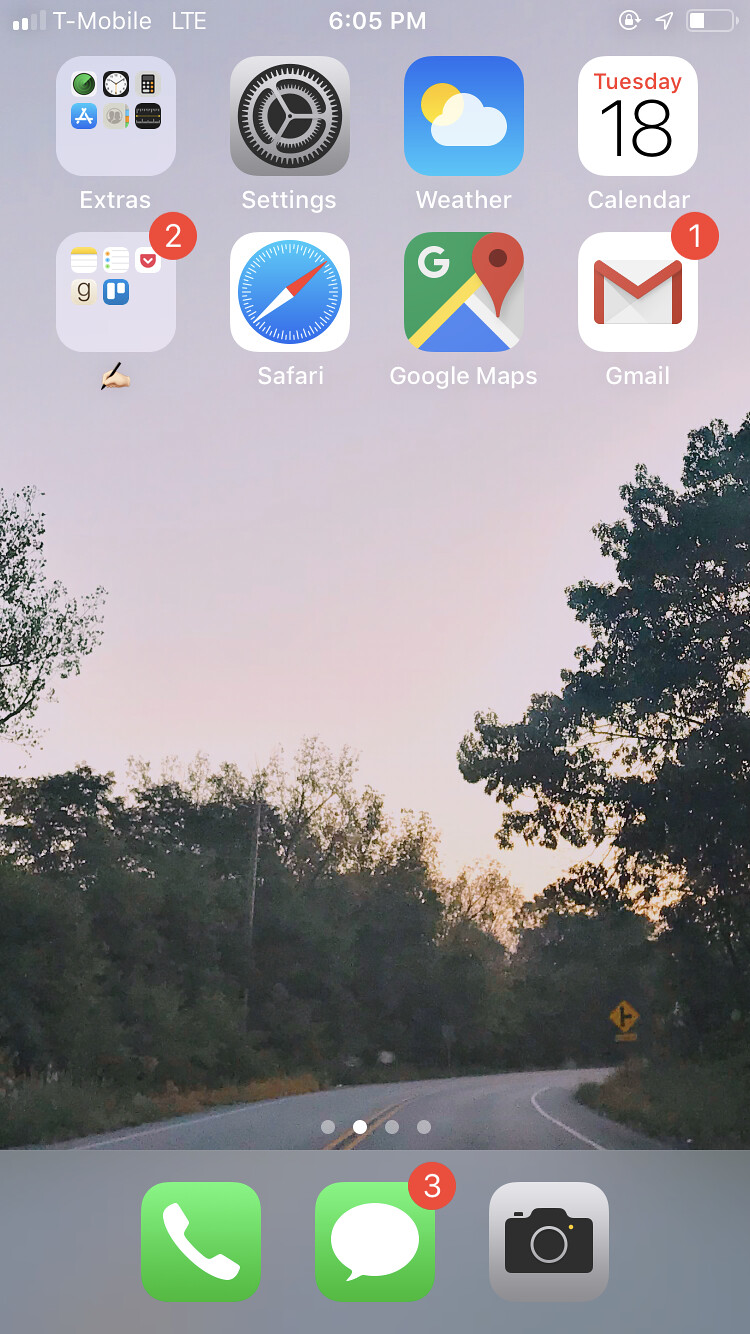A detailed screenshot of a smartphone's home screen is displayed, showcasing a variety of icons and a scenic background. In the top left corner, the T-Mobile logo is visible, while the top right corner features the battery icon indicating the remaining battery life. Centered at the top in white text is the current time, 6:05 p.m.

The home screen features a grid of icons arranged in two rows. The first row consists of four icons:

1. A folder labeled 'Extras' contains six icons.
2. The settings icon, depicted as a metallic gear.
3. The weather app, illustrated with a blue gradient background featuring a sun and a cloud.
4. The calendar app icon, primarily white with 'Tuesday' in red text at the top and '18' in large black text, taking up most of the space.

The second row also has four icons:

1. Another folder, labeled with an emoji of a hand holding a pencil, containing five icons.
2. The Safari web browser icon, represented by a blue compass.
3. The Google Maps icon, a close-up of intersecting streets with a red map pin.
4. The Gmail icon, shown as a white envelope with red edges.

The background image is a picturesque highway scene flanked by dense woods. A yellow road sign is visible on the left side of the road. The photograph captures a dusk setting, with a dark blue sky at the top fading into a yellow-orange hue near the horizon behind the treeline.

At the bottom of the screen are three primary app icons:

1. The phone app, represented by a green square with a white telephone icon.
2. The messaging app, depicted as a white speech bubble on a green background, with a red circle in the top right corner indicating three unread messages.
3. The camera app, illustrated by a gray button with a black camera icon.

Overall, the screenshot provides a clear and detailed overview of the phone's home screen layout and features.